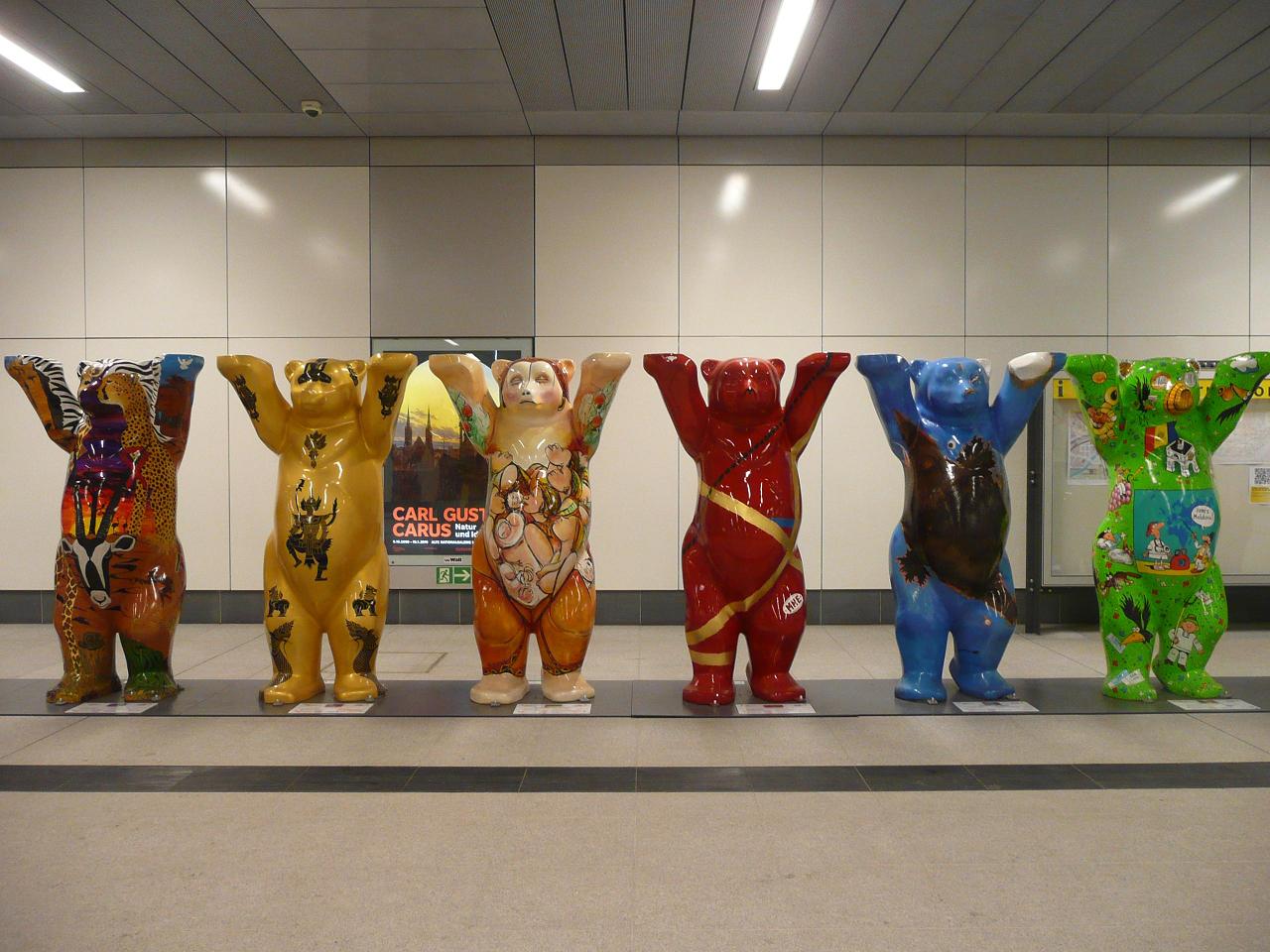This image captures an art exhibit located in what appears to be a clean, well-lit subway station or an airport terminal. The setting features a gray-tiled ceiling with overhead lighting, a tan-colored floor, and mostly white and gray tiles on the walls. There's a noticeable LED sign in the background that reads "Carl Gust Kares." The main focus of the image is a line of six colorful, uniquely painted bear sculptures, each standing on its hind legs with its paws raised above its head.

1. The first bear exhibits an African safari theme with animal prints and designs, including a cheetah face, zebra stripes, an antelope on its belly, and giraffe patterns on its legs. It also features a blue paw with a bird on it and a zebra-patterned paw.
   
2. The second bear is predominantly yellow with Chinese symbols and tribal motifs. Its design includes Chinese dragons on its legs and various symbols on its head, chest, and the underside of its arms.
   
3. The third bear features a serene, meditative theme with paintings of people, mostly women, and floral patterns on its arms. The figures have their heads raised, and the overall ambiance suggests calmness, possibly akin to yoga.
   
4. The fourth bear is striking red with a gold ribbon-like design and a black dotted line wrapping around its body, creating dynamic, intersecting patterns.
   
5. The fifth bear is blue with a broad brown design across its chest that might depict a bird or a turtle. Its left ear and paw are white, providing stark contrast.
   
6. The sixth and final bear is vibrant green with a whimsical, cartoonish design. It features a comic strip in the middle with various elements, including the Eiffel Tower, a flying blackbird carrying mail, a dreaming cat, and other playful characters.

Together, these bears showcase a diverse range of artistic styles and cultural motifs, creating an eye-catching display amid the sterile backdrop of the station.